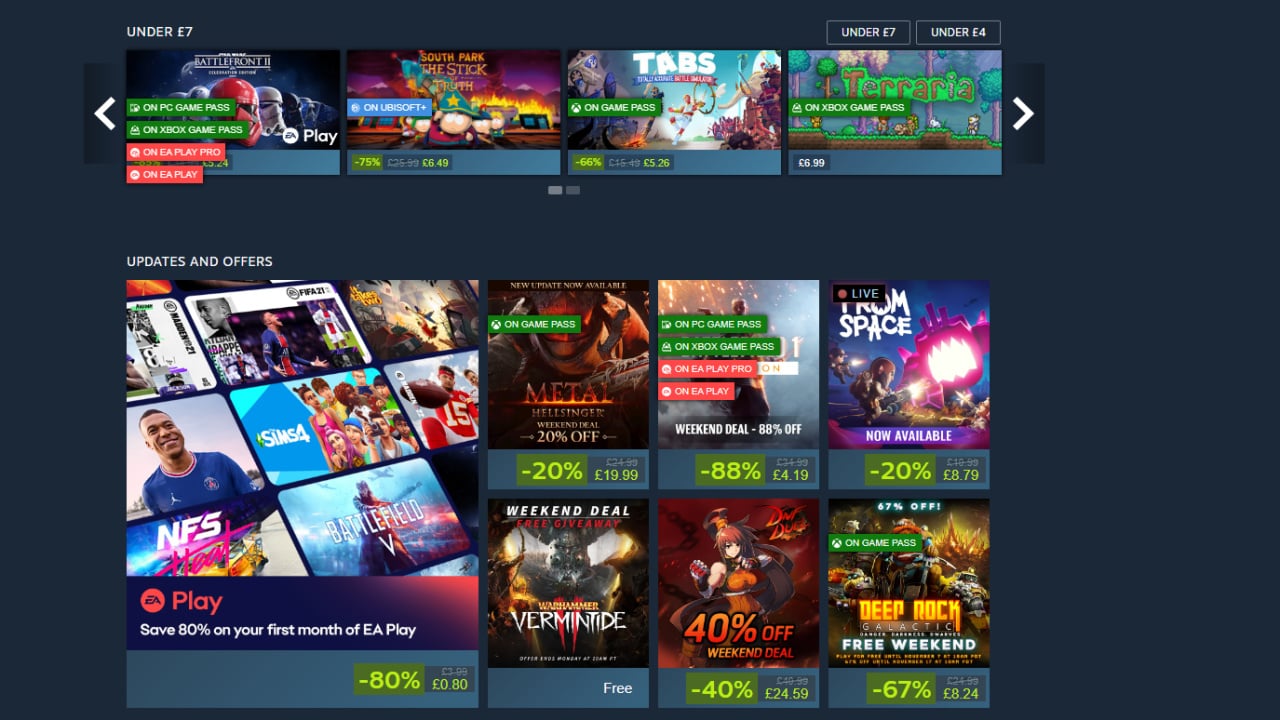The image depicts a screenshot from a device showcasing a digital store or application platform, primarily focusing on available games. The background is a deep gray, almost black shade, which serves to highlight the text and images prominently. At the very top, in white print, the text reads "Under £7," indicating budget-friendly game options.

The screen is segmented into different sections. The upper portion displays a game titled "Battlefront II," accompanied by the "EA Play" logo. Notably, on the left side of this section, there are green labels indicating game accessibility: "On PC Game Pass" and "On Xbox Game Pass," both highlighted in green boxes with white text.

Further down, there is a light red box labeled "On EA Play Pro," suggesting additional subscription-based access. The visual layout presents four game title images in the top row. Below this main section, there are labels and icons such as "Updates and Offers" in white text, signifying additional content or deals.

In the middle and bottom sections, there are six more game title images, organized in two rows of three. Some of these games have discount tags, such as "80% off" or "88% off," making them particularly eye-catching for bargain hunters. The detailed arrangement and color-coded labels offer a clear and organized browsing experience for users looking to explore new game options.